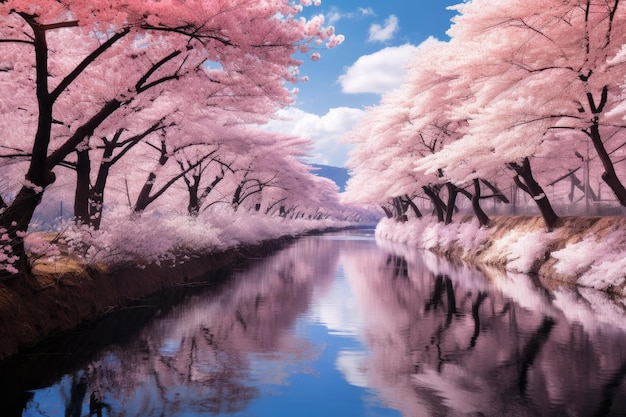This vibrant and detailed photograph captures a serene, picturesque scene of a stream flowing down the center, flanked by rows of stunning cherry trees in full bloom. The tall cherry trees, with their dark trunks and stunning pink blossoms, form an almost arch-like canopy over the water, creating a dreamy, cloud-like effect. Smaller shrubs with pink floral details add to the scenic beauty beneath the larger trees. The calm water perfectly mirrors the pink blossoms and the lightly rippled reflections of the trees, extending far into the distance. Above, a bright blue sky with billowing white clouds enhances the tranquil atmosphere. There are no people, animals, or buildings in the image, allowing nature's beauty to take the center stage.